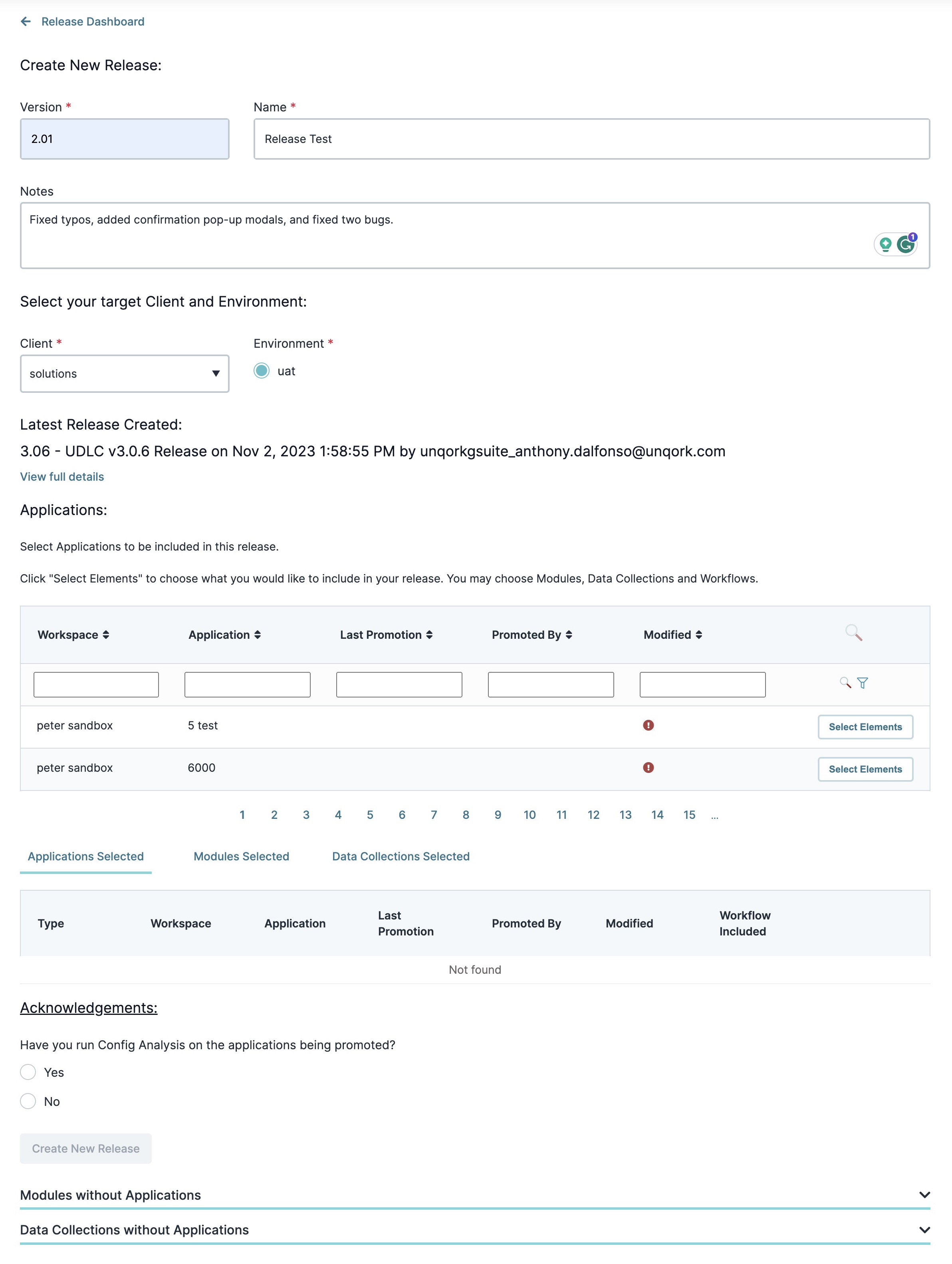The image depicts a detailed **Release Dashboard** interface. At the top, the title "Release Dashboard" is prominently displayed. Below that, there is a section labeled "Create New Release," featuring a form to fill out essential release details. 

- **Version:** 2.01
- **Name:** Release Test
- **Notes:** 
  - Fixed Typos
  - Added Confirmation Pop-up Modals (M-O-D-A-L-S)
  - Hold Alls
  - Fixed Debugs

The next section is about selecting the target client environment, currently set to **UAT Environment**. The associated solution is labeled "Clients."

Underneath, there's a historical record titled **Latest Release Created**, showing details of the most recent release:
- **Version:** 3.0.6
- **Date:** November 2, 2023

Adjacent to this, details of the applications involved are provided.

The following section is a smaller form for inputting workspace details:
- **Application:** [Dropdown Field]
- **Last Promotion:** [Date Field]
- **Promoted By:** [Text Field]
- **Modified:** [Text Field]

Additional details include:
- **Application Selected**
- **Module Selected**
- **Data Collection Selected**

Each requires the user to specify:
- **Type**
- **Workspace**
- **Application**

An acknowledgment section asks if the user has run a Configuration Analysis, offering "Yes" or "No" options.

Finally, two expandable sections list:
1. **Modules Without Applications**
2. **Data Collection Without Applications**

These sections feature clickable arrows to expand for more detailed information.